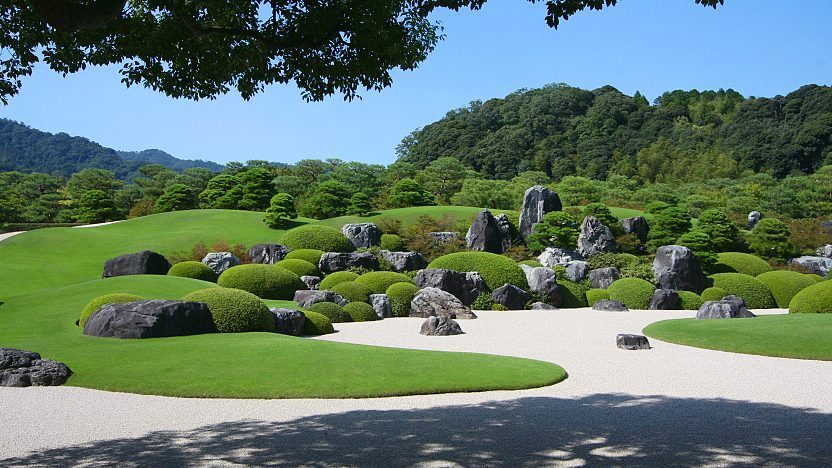This horizontal rectangular photograph captures a meticulously landscaped, meditative park with a reflective garden. In the foreground, a sidewalk diverges in multiple directions, curving gracefully and winding around the scene. The sidewalk approaches a rock garden filled with large boulders, bushes, and fine white stones that evoke a serene and manicured Japanese-style garden. This area transitions into a circular courtyard-like section surrounded by gently rolling, man-made hills and small, neatly trimmed round bushes. The grass throughout the park is impeccably maintained, reminiscent of a golf course's pristine condition. Above, branches of a tall tree cast intricate shadows onto the concrete and gravel paths below. The background features a line of tall trees with lush green leaves, extending towards distant hills or mountains also covered with verdant foliage, all set against a clear, light blue sky free of clouds. The overall scene creates a harmonious blend of natural and designed beauty, ideal for peaceful contemplation.